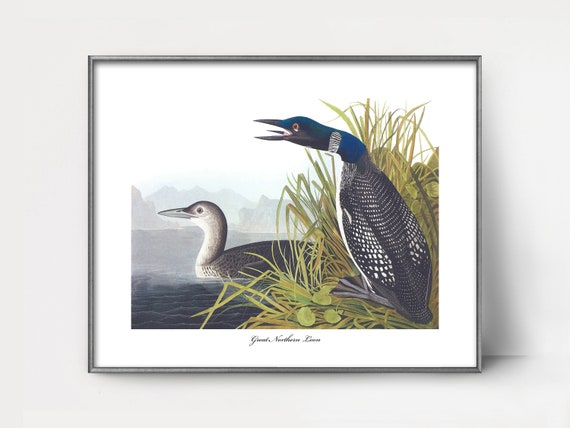The image portrays a print of two ducks set within a thin, gray metal frame. The artwork, whether hand-drawn or digital, presents one duck with a vibrant, sapphire blue head and white and dark blue feathers, situated in a grassy marsh setting. This duck appears to be making a call with its mouth open and tongue visible. Adjacent to it, a more subdued gray and silver duck with a white neck swims in the water. The background features a serene landscape with mountains, while the top fades to white, blending seamlessly with the mat surrounding the print. The text at the bottom reads "Great Northern," although the last word is difficult to discern.